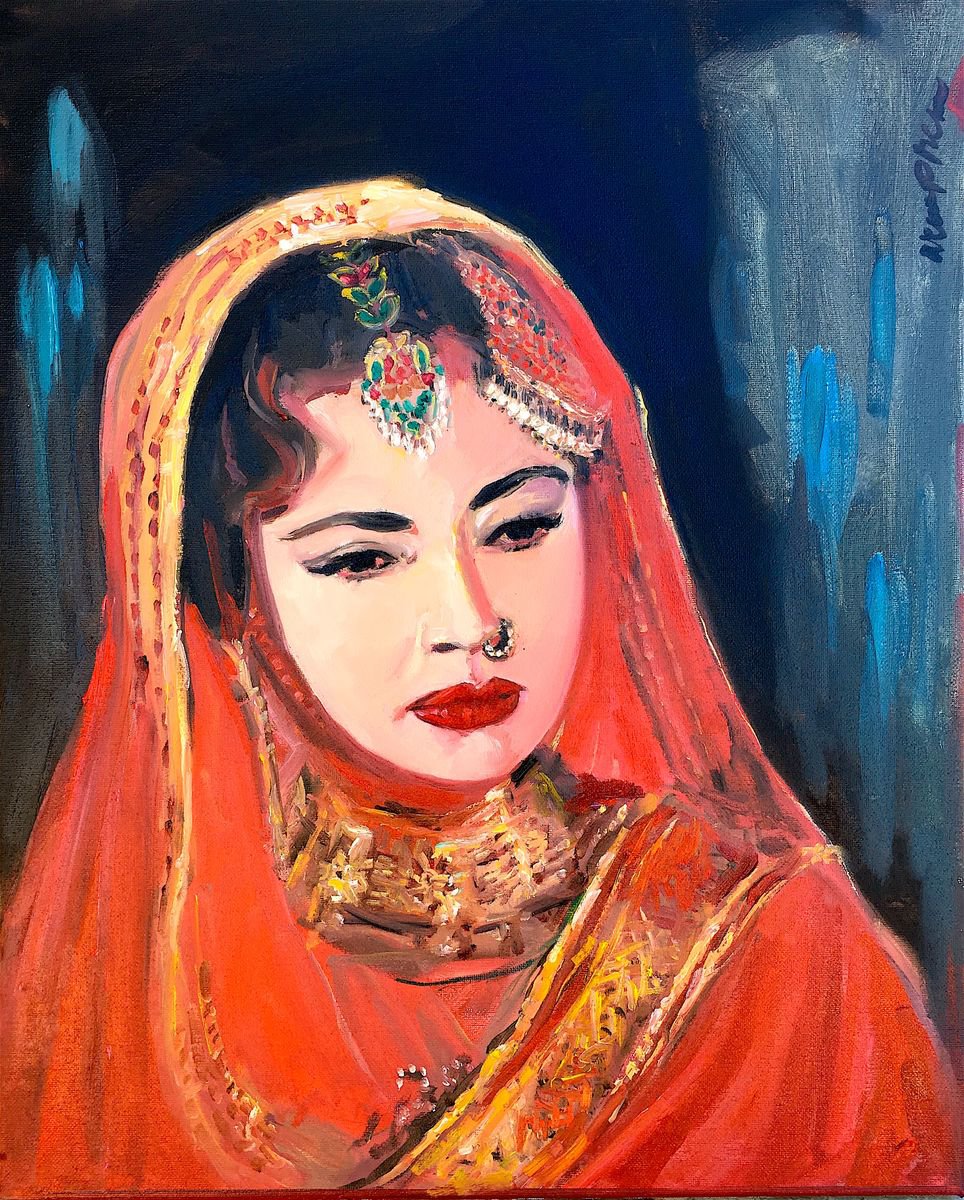The image is a detailed painting of an Indian bride, showcasing rich cultural attire and jewelry. The woman, slightly left of center, faces to the right with a straight expression. Her ensemble includes an intricate red sari adorned with gold trim and patterns along its edges, as well as a hood over her head that features red sequins and gold accents. She wears a prominent gold choker around her neck, red lipstick, and has dark black hair and eyebrows. Her forehead is decorated with hanging jewels that extend from the middle up over the back of her head and under the hood, with additional decorative elements visible on the left side of her forehead. She also has a nose ring in her left nostril. The visible part of her body is from the chest up. The background varies from navy blue to lighter shades of blue with hints of gray, creating a serene backdrop. In the upper right corner of the painting, there appears to be a signature in black, likely indicating the artist.